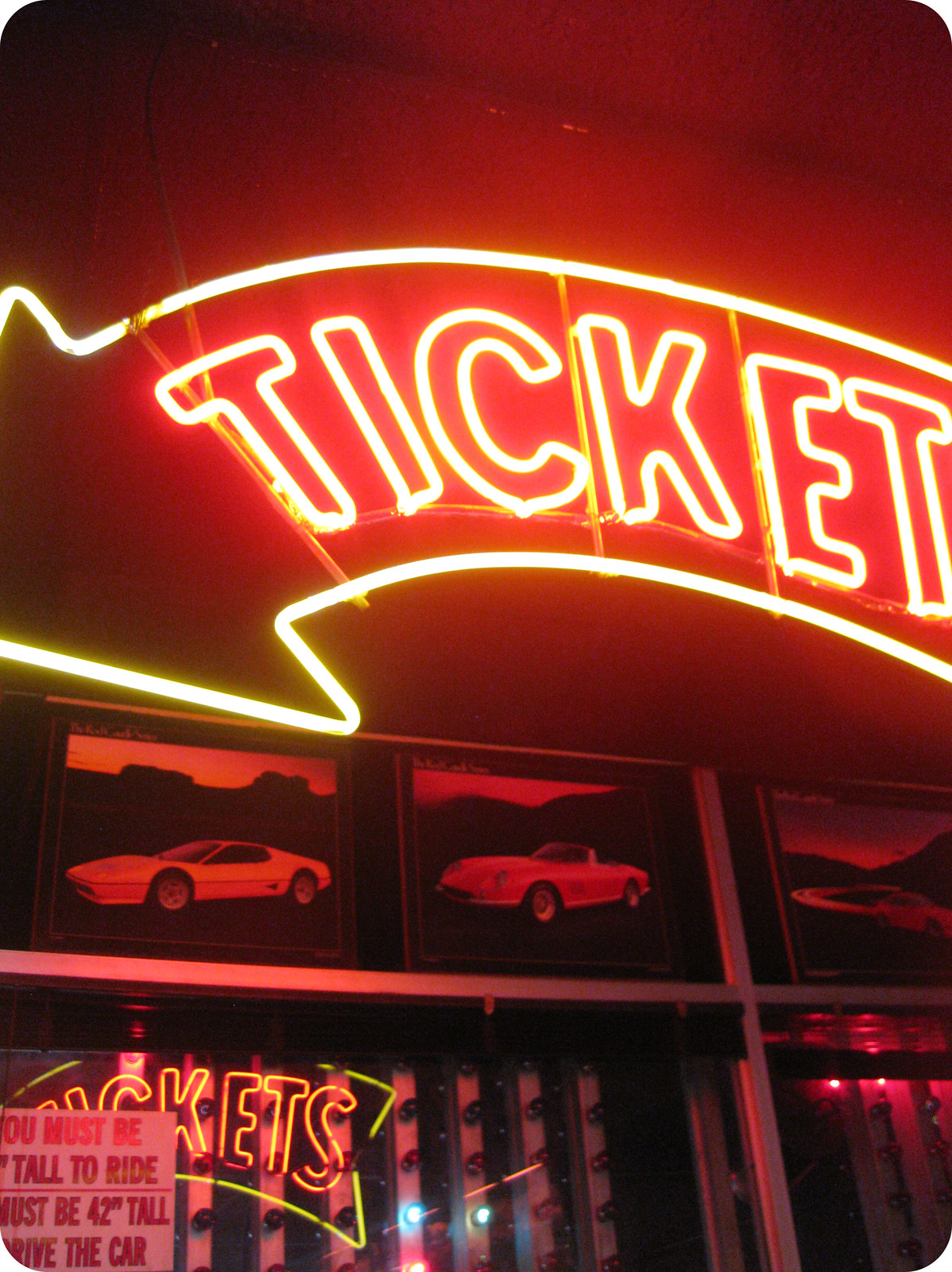This photograph captures a vibrant, nostalgic scene inside an arcade or fair. Dominating the upper part of the image, a large neon sign in a glowing, curved arrow shape points downward and to the left, with the word "TICKETS" illuminated in eye-catching yellow. This sign contrasts against a red wall, creating a warm and inviting ambiance. Directly below the sign, bathed in the orange glow, are framed photographs of sleek sports cars, likely exotic models from the 70s and 80s, emphasizing a vintage charm.

Below these photos, a glass window, possibly part of a ticket booth, features another neon sign or its reflection, repeating the "TICKETS" message. On this glass, a sign informs guests that they must be 42 inches tall to participate in a car ride or attraction. Adding to the festive scene, colorful carnival lights twinkle in the background, enhancing the overall lively atmosphere. Although the image doesn't include people or show the ride itself, the details suggest this is a ticketing area for a car-themed exhibit or ride at an amusement park or fair.